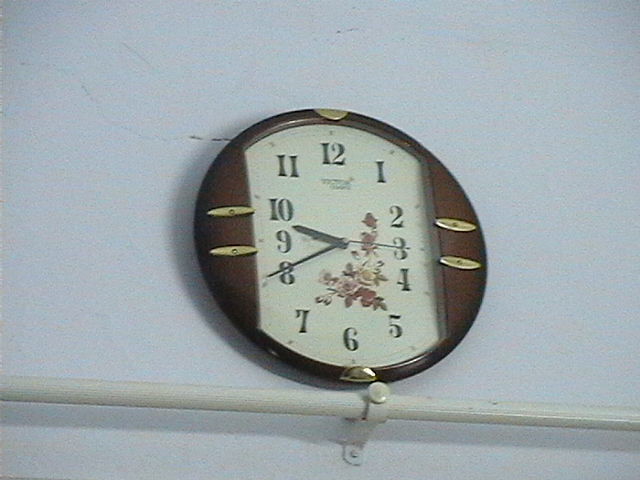The image showcases a clock prominently displayed on a smooth white wall. The clock is circular with a distinguished brown border that features straight lines on the left and right, converging into the circular shape. Below the clock, a beige cylindrical curtain rod is affixed to the wall. The clock face is a soft off-white, adorned with black numerals ranging from 1 to 12. There appears to be a subtle floral design embellishing the clock face, adding an elegant touch. The clock is equipped with black hour, minute, and second hands, and it precisely indicates the time as 9:40 and 15 seconds. Additionally, there are gold-colored attachments positioned at the top, bottom, left, and right sides of the clock, contributing to its ornate appearance.